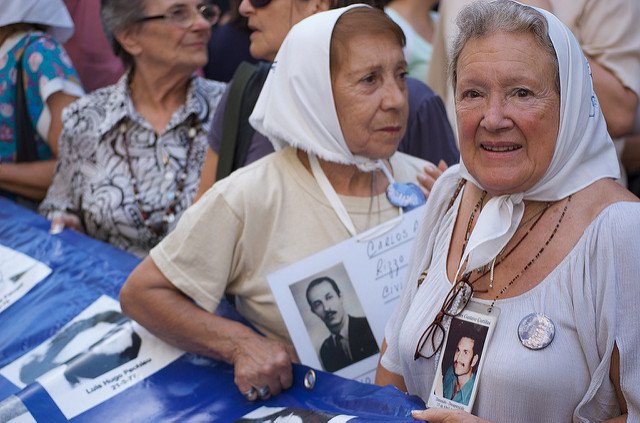This color photograph depicts a poignant scene of elderly women gathered at what appears to be a memorial service or possibly a protest. These women, appearing to be in their late 60s to early 70s, are honoring deceased loved ones, likely men, as they hold banners and photographs with names and dates. 

In the foreground, two women stand out. The woman on the right, with gray hair and rosy cheeks, gazes pensively into the camera. She wears a white headscarf and a light gauze blouse, with a pair of glasses hanging around her neck from a lanyard. She also has a laminated photograph of a man, presumably a lost loved one, hanging around her neck, along with a shiny silver button with foreign writing pinned over her right breast.

Next to her, on the left, another woman, also donning a white headscarf, looks pensively to the side. She wears a piece of paper around her neck attached with a white ribbon, featuring a black and white photo of a man and the visible name "Carlos A. Rizzo," suggesting a Spanish background. 

They stand in front of a blue shiny cloth banner, which is adorned with numerous photographs of other individuals, further indicating this event's somber nature. The setting is outdoors, in the daytime, enhancing the scene's powerful atmosphere of remembrance and possibly a collective search for missing loved ones.